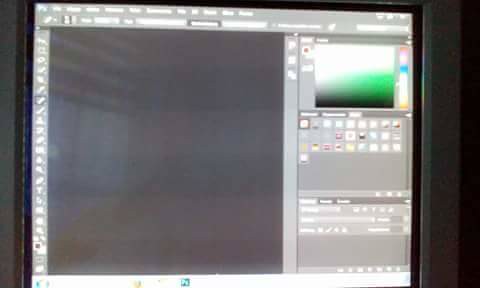This photograph captures a close-up of a square computer monitor featuring a black bezel. The visible screen displays an application for painting or drawing, framed by a grey border. A Windows taskbar, potentially from an older version of Windows, is present at the bottom. On the right side of the application interface, there's a color palette selector currently highlighting various shades of green, ranging from white and green to black. Notably, the center of the application screen shows no open document or active canvas. The details behind the monitor remain indistinguishable in the image.